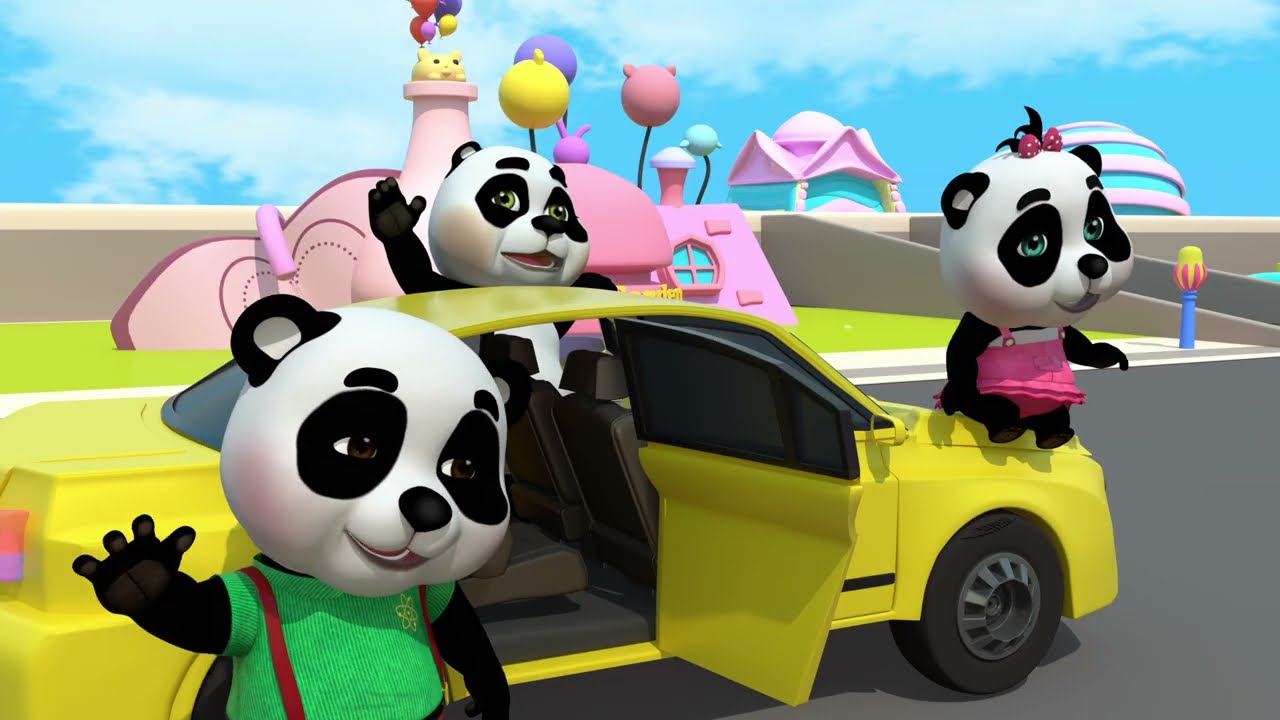The digital artwork depicts a vibrant, cartoonish street scene featuring three animated pandas around a yellow car. The car, a four-door vehicle with black-tinted windows and an open rear passenger door, stands prominently in the foreground of the image. To the left, a boy panda with black circles around his eyes, black ears, and a green shirt with red suspenders is waving his left paw, while his right paw is held close to his body.

Perched on the hood of the car is a girl panda adorned with a pink dress, frills at the bottom, and a pink bow with white polka dots tied around a sparse sprig of hair on her head. She appears to be getting off the hood, moving towards the right side of the image.

Standing behind the car and waving with his left paw is an adult panda, larger than the other two, with no clothing. This family tableau is set against a backdrop of whimsical, pink cartoon buildings. The nearest house has a butterfly-esque design and is equipped with a steeple and windows, while other structures include additional pink homes and a castle-like building with spires. The sky above is cartoonishly blue with clouds, dotted with colorful balloons in shades of yellow, purple, and reddish pink. A paved street runs through the scene, framed by a sidewalk and grassy patches, completing the lively and playful setting.